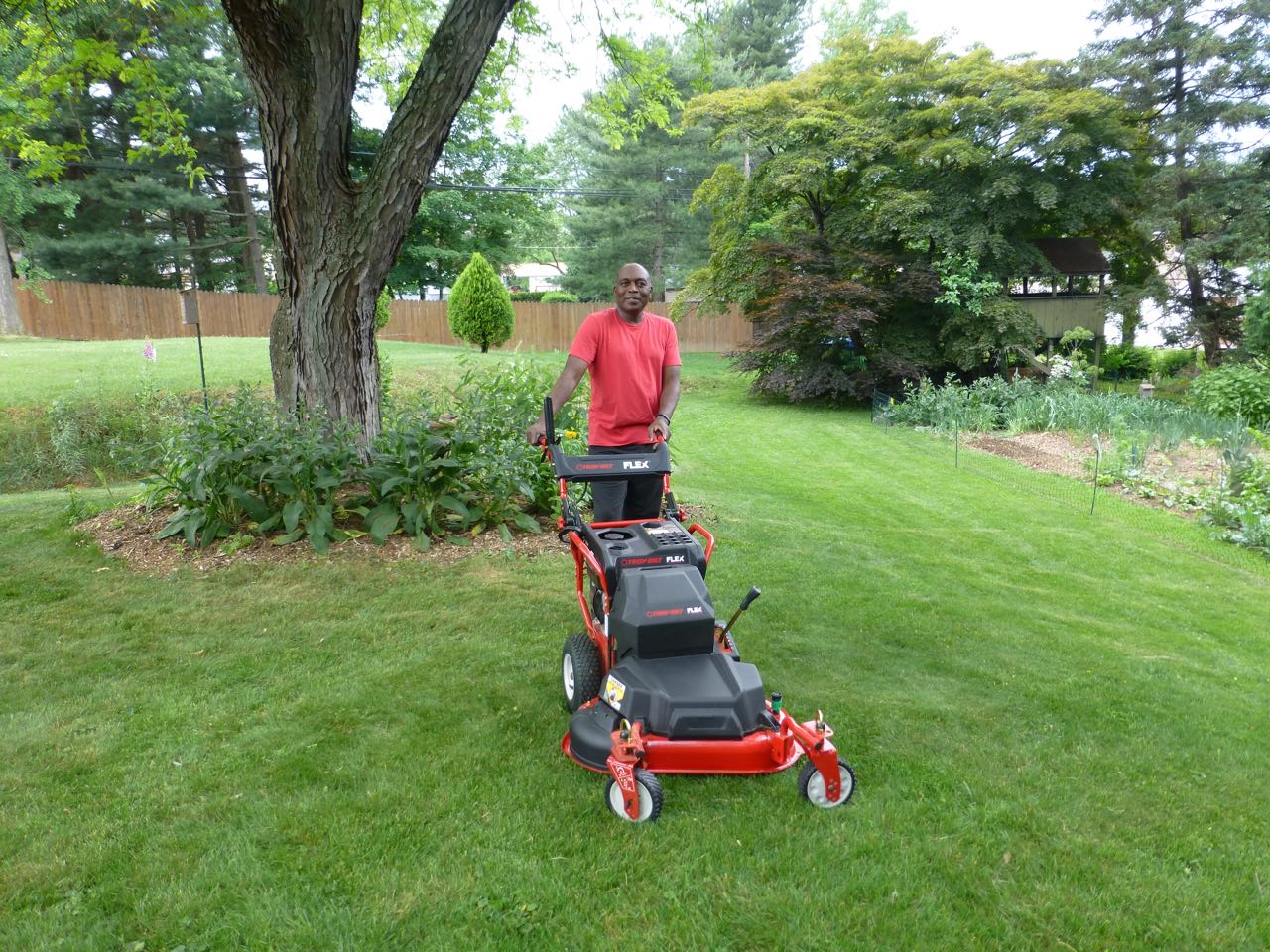In this image, an immaculate, sprawling lawn is prominently featured, with its rich green grass meticulously maintained. Standing proudly amidst this verdant expanse is a gentleman wearing a red shirt and black slacks or shorts indistinguishable from the angle. He operates a large, zero-turn mower designed for standing operation, allowing for precision mowing across the uneven, terraced landscape. A prominent tree, encircled by well-maintained mulched plants, stands behind him, adding a touch of natural elegance to the scene. The terrain appears to slope in multiple directions, creating a dynamic, rolling effect. The gentleman, smiling contentedly, seems pleased with his work, suggesting a sense of pride, whether he owns the lawn or is tending it professionally. In the distance, the lawn gently slopes towards a suspected vegetable garden, adding to the overall idyllic setting. The sky above is overcast, casting a soft light over the scene, enhancing the lush greenery without the harshness of direct sunlight.